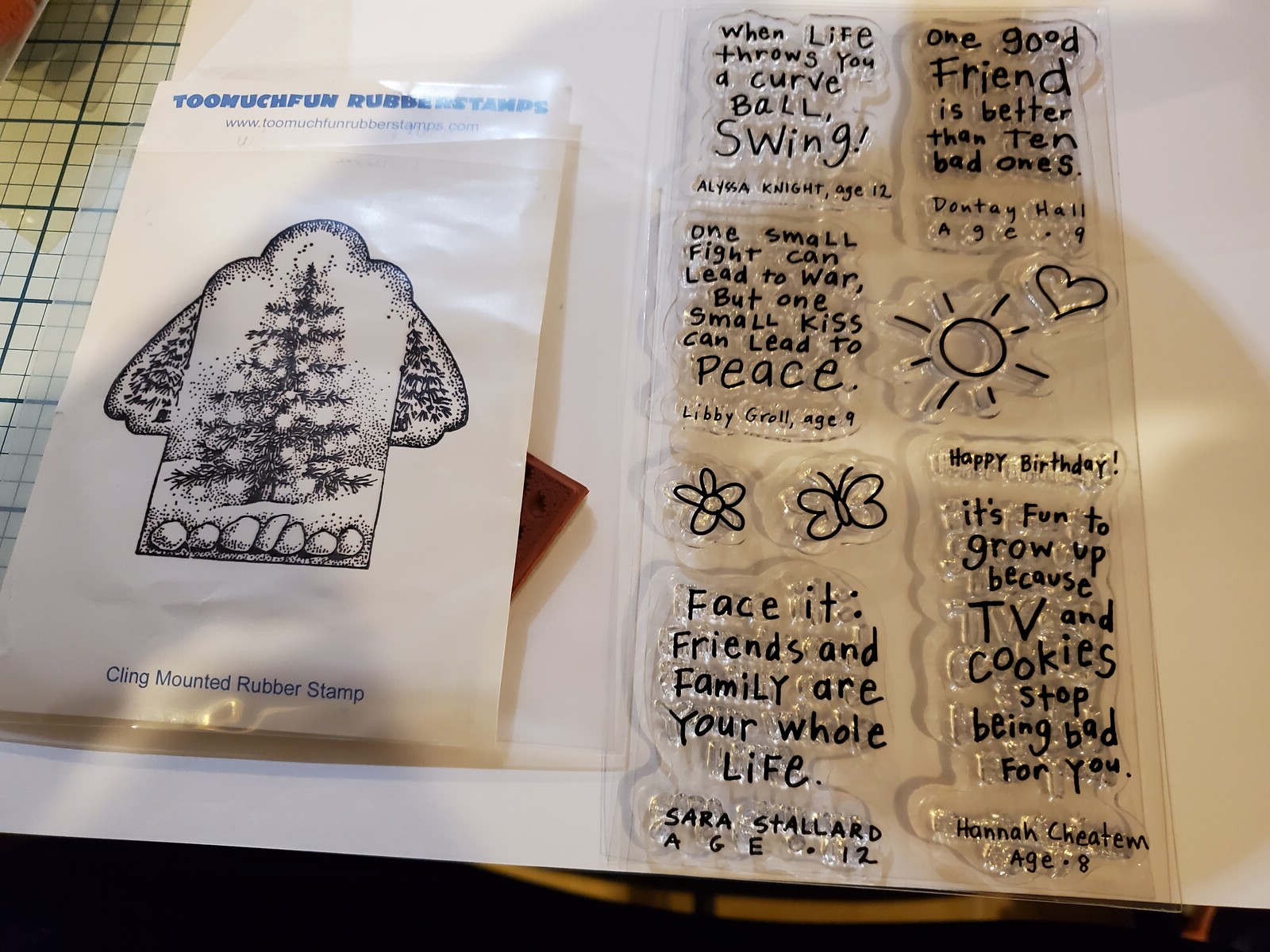The photograph captures a work table displaying an assortment of arts and craft supplies. On the left side, a white package is prominently featured, labeled "Too Much Fun Rubber Stamps, Cling Mounted Rubber Stamp" in blue font at the top and bottom. This package appears to contain a rubber stamp, possibly with a Christmas theme. To the right of the package, there are various clear plastic stencils with curvy, intricate designs. These stencils feature stamped messages, such as "When life throws you a curveball, swing," "One good friend is better than ten bad ones," "One small fight can lead to war, but one small kiss can lead to peace," and "Face it, friends and family are your whole life." Additionally, the stencils include shapes like a heart, a sunflower, and butterflies, along with celebratory messages such as "Happy Birthday" and "It's fun to grow up because TV and cookies stop being bad for you." The overall arrangement is set against a large piece of white construction paper, providing a clear and organized backdrop for the items displayed.